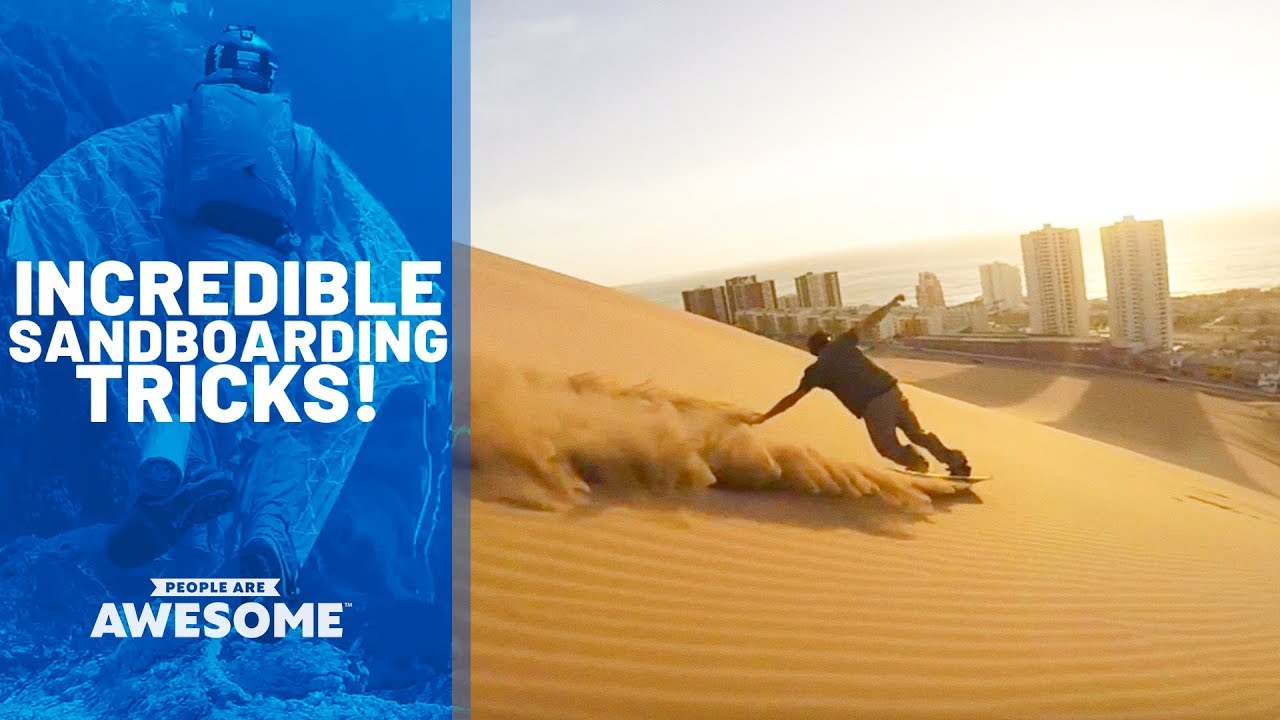The image is an advertisement for sandboarding and extreme sports, displayed as a composite of two main visuals set against contrasting backgrounds. On the right, a young man dressed in brown is captured in dynamic motion, sandboarding down a large dune at high speed. His left arm touches the sand to balance, while his right arm reaches upward, kicking up a spray of sand. The scene is set in a vast desert with predominantly sepia tones, and in the background, a cityscape with numerous tall buildings is visible, hinting that the location might be in India or the Middle East.

On the left side, overlaid on a blue background, is an infographic illustrating a person in a wingsuit, emphasizing another extreme sport. The text over this section reads "Incredible Sandboarding Tricks!" and at the bottom, "People are Awesome!" This thorough depiction showcases the thrill and diversity of the extreme sports being promoted.